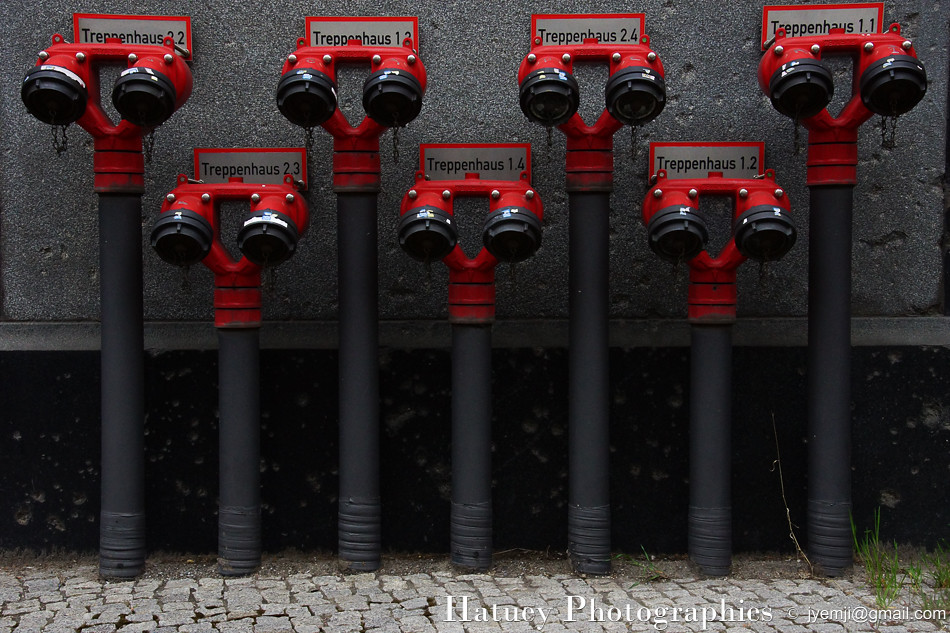This photograph, labeled "Halney Photographics," features a setting with a distinctly rocky floor composed of flat stones tightly fitted together. Emerging from this rocky surface are seven black pipes arranged alternately in height—four tall and three shorter ones. The pipes are symmetrical and resemble industrial installations. At the top of each pipe, there is a red unit with two extensions capped in black, resembling binocular lenses. Each pipe has the word "Treppenhaus" inscribed on it along with unique numerical identifiers ranging from 1.1 to 2.4. The background is dominated by a solid gray brick wall. The photo also contains a watermark or contact information which includes an email address, jjyemi@gmail.com, at the bottom of the image.